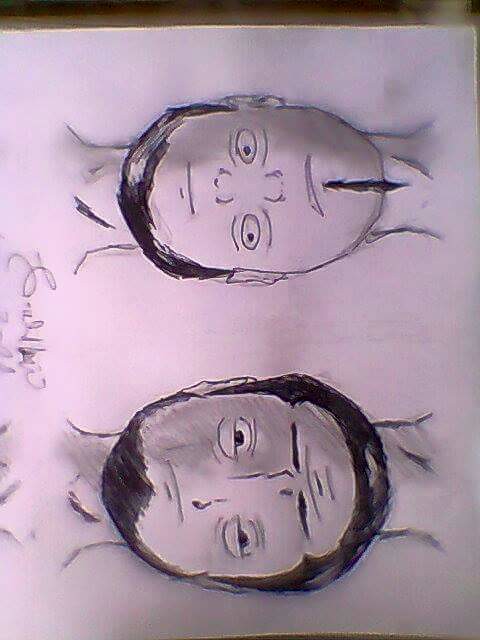The image displays a piece of white paper, positioned slightly askew, featuring two intricately illustrated male faces. These portraits, rendered in either pencil or charcoal, exhibit an artistic duality, appearing as complete faces regardless of whether they are viewed right side up or upside down.

The upper drawing reveals a face divided into two distinctive styles. On one side, the man has a full head of hair or a beard, while the opposing side showcases a mohawk or a soul patch, ingeniously crafted to merge seamlessly into a coherent face from either angle.

Beneath this, the lower illustration depicts a man sporting a full beard, designed to create the illusion of a man with both a full head of hair and a beard, no matter the orientation of the paper.

Together, these imaginative drawings highlight the artist's skill in creating reversible and multifaceted portraits on a simple sheet of paper.